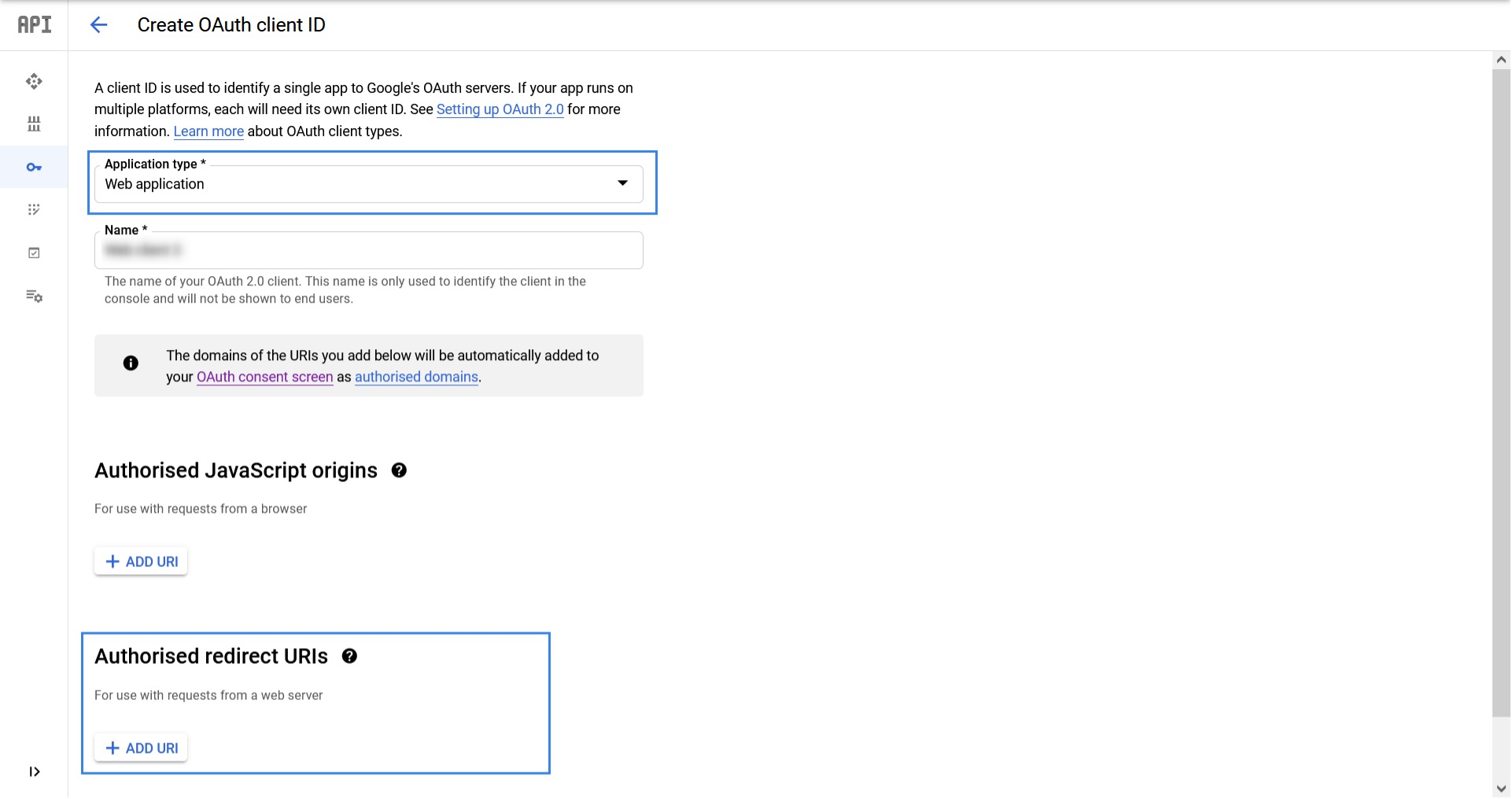This portrait-oriented screenshot from a laptop or computer displays an API management interface. The screen is approximately one and a half to two times wider than it is tall and features a thin gray border along the top edge.

About 5-10% down from the top, another thin gray line divides the screen, creating a header section. The header prominently shows the label "API" in dark black font. Underneath this header, six icons are displayed, with the third icon, depicting a key, highlighted in blue with a blue box around it, indicating selection. To the right of the "API" header, there is a backward-pointing arrow in blue, followed by the text "Create OAuth client ID".

Below the header, there is a black-font paragraph providing instructions, succeeded by a gray rectangular horizontal box. This box has a black header labeled "Application Type" with an asterisk next to it, denoting a required field. The selected option here is "Web Application", indicated by a blue-highlighted drop-down caret on the right.

Subsequent to this, there's another section labeled "Name", which contains some placeholder text in gray. Below this, a gray box features black font and an information icon, which precedes the black header "Authorized JavaScript Origins". Beneath this header, a white box with blue font instructs the user to "Add URI".

Lastly, there is another section labeled "Authorized Redirect URIs", surrounded by a horizontal blue rectangular box. This section is intended for the entry of redirect URIs authorized for the application.

Overall, the interface seems to be guiding the user through the setup of OAuth client ID parameters for a web application.